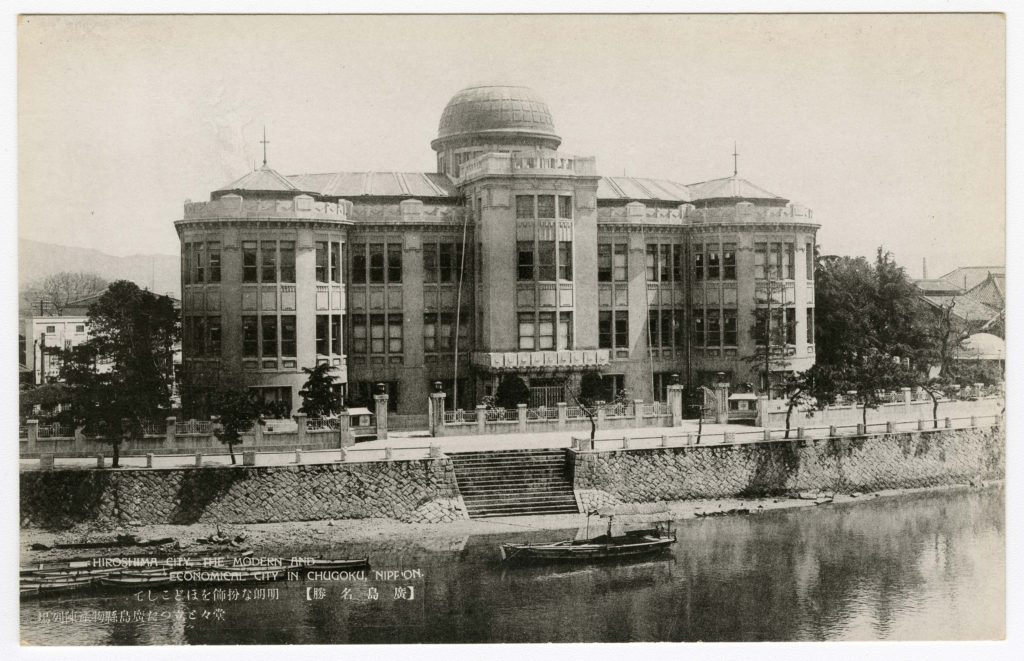This black-and-white photograph captures a stately, three-story building prominently situated along a riverfront. The central architectural feature is a rounded turret or domed roof. In front of the building, which resembles an office or government structure, lies a stone fence with columns and a staircase flanked by stone walls, leading directly to the waterway. A small boat is visible at the base of the stairs, with additional boats or canoes faintly seen in the bottom left corner, partially obscured by white text. The inscription reads, "Hiroshima City, the modern and economical city," accompanied by Japanese characters. The setting is serene, underscored by the absence of people, and enhanced by the presence of trees surrounding the building and other distant structures. Far off in the background, a mountain or hill looms, completing the tranquil scenery of this historical riverfront.